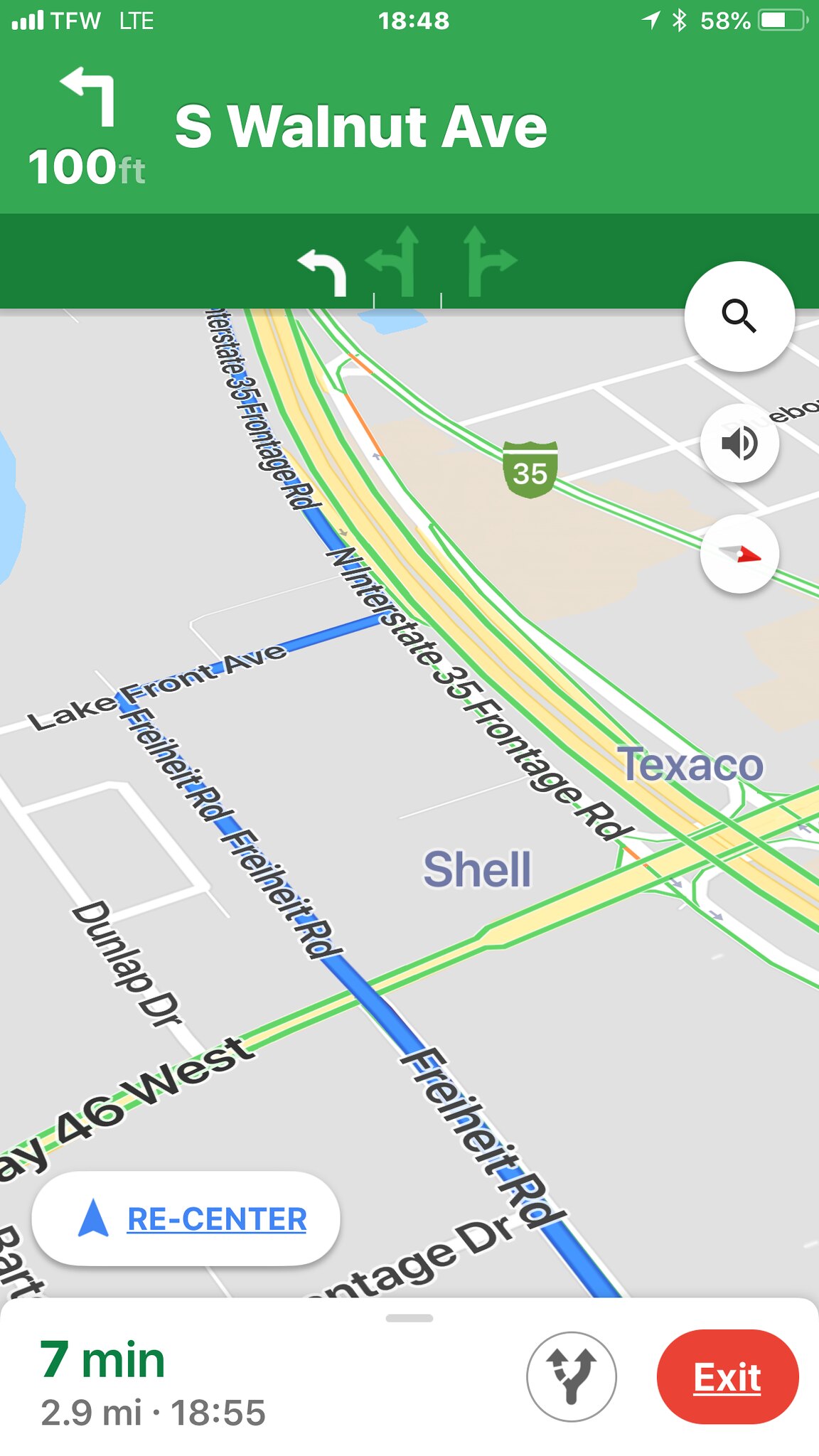This screenshot, taken on an iPhone as indicated by the battery icon at the top right corner showing a 58% charge, captures a detailed view of a navigation map. The status bar displays various symbols: Bluetooth, location, the time set on a 24-hour clock reading 18:48, and the carrier name "TFW" alongside LTE signal bars on the left side. The map itself focuses on a route, advising the user to make a left turn onto South Walnut Avenue in approximately 100 feet. The final destination is noted to be seven minutes away from the current location.